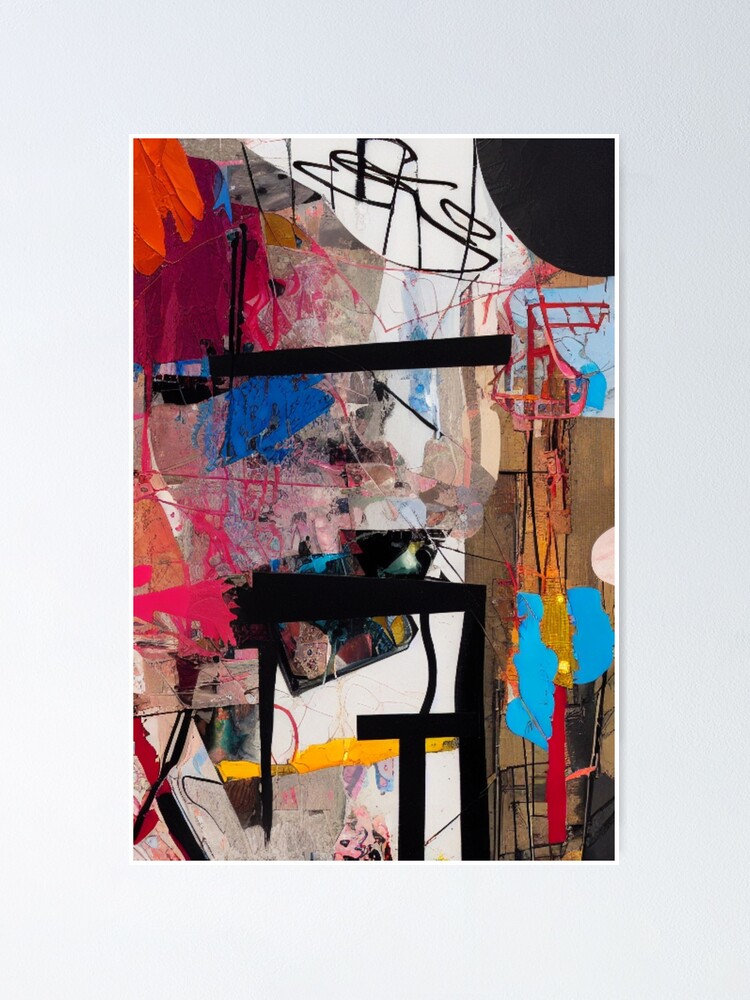The image showcases an abstract painting, matted on a white piece of paper and framed by a gray border, possibly the photograph’s background. The artwork features an eclectic array of colors and shapes with no distinct identifiable forms, creating an enigmatic and colorful tapestry. Dominant colors include black, red, blue, yellow, brown, and various warmer hues like orange and magenta. Notably, there is a prominent black half-sphere in the upper right corner and a smattering of black splatter marks across the canvas. The painting appears to depict a central black object, reminiscent of a table, with a bowl-like shape on top, surrounded by a chaotic mix of splatters. The abstract nature of this piece, rich with complex patterns and vibrant colors, invites myriad interpretations and evokes a sense of creative disarray.